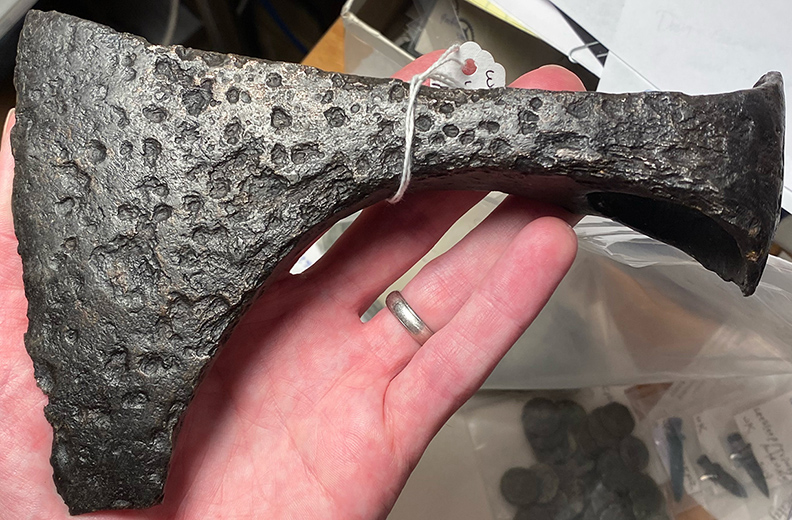This color close-up photo captures a Caucasian left hand, adorned with a silver wedding band on the ring finger, holding a dark iron-colored object. The object, possibly an ancient axe head, exhibits clear pitting and divots throughout its structure, with some areas reflecting the flash, indicating a metallic composition. A paper price tag, attached with a piece of string, loops around the handle of the axe head, though the writing is obscured from view. In the bottom part of the image, there's a plastic bag that appears to contain papers and perhaps some black circular objects or coins, suggesting the bag might have housed the axe head previously.